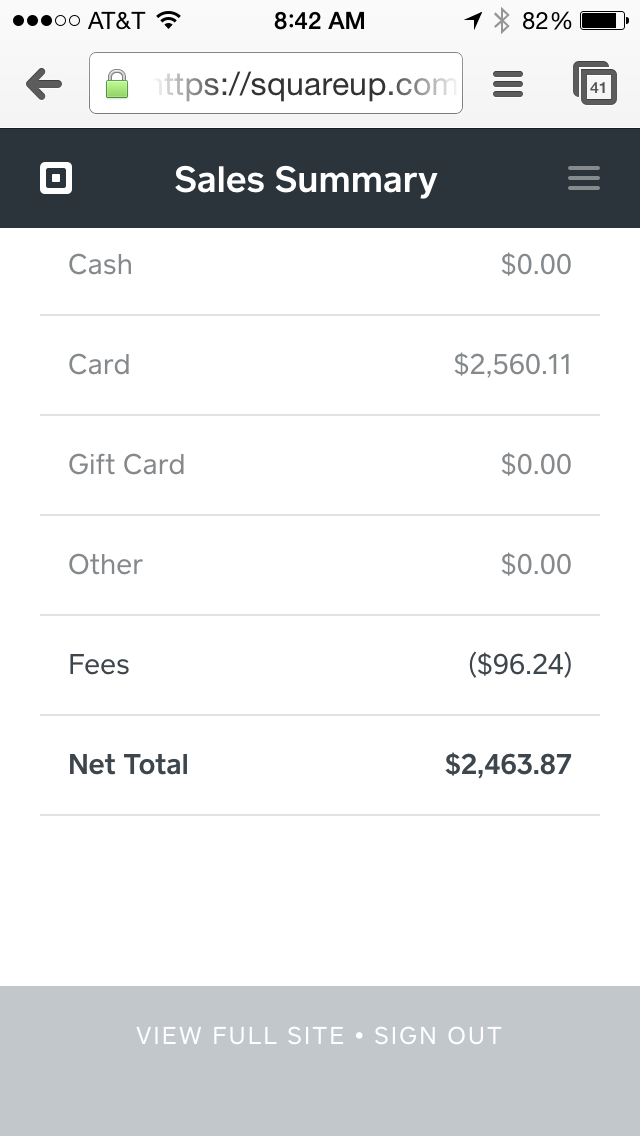The image is a screenshot taken from an older mobile device, likely a smartphone, evidenced by the presence of signal strength indicators, an AT&T provider tag, the time (8:42 AM), and an 82% battery icon at the top of the screen. The URL, partially visible, is "https://squareup.com". Below the URL, a blue banner with white text reads "Sales Summary." The page consists of multiple white sections separated by gray lines, featuring semi-gray text and numbers. The sales summary details are as follows: Cash: $0, Card: $2,560.11, Gift Card: $0, Other: $0, Fees: $96.24, and Net Total: $2,463.87. At the bottom of the screenshot, there is a gray bar displaying options to "View Full Site" and "Sign Out." The web page's rudimentary design suggests it might not be from a modern mobile interface.